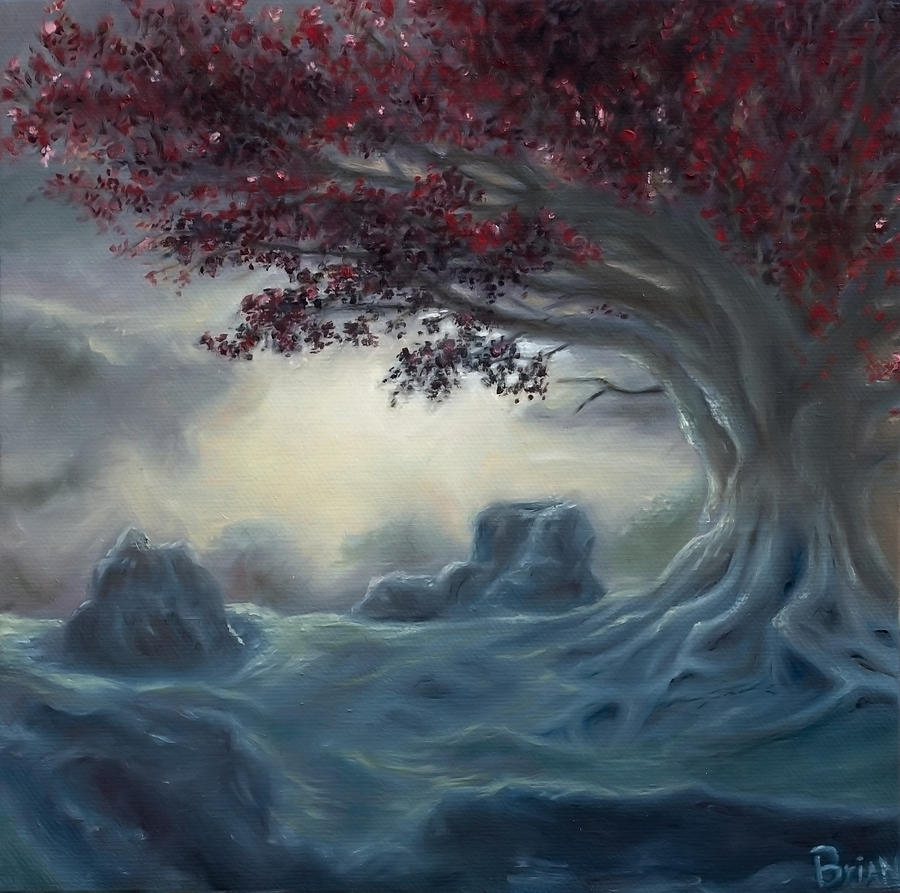This square oil painting, signed "Brian" in light blue text at the bottom right-hand corner, captures a dramatic nighttime or early dawn scene. At its core, a sprawling tree dominates the canvas, rooted on a cliff or mountaintop. The tree’s thick, gnarled roots anchor it firmly into the ground, which is primarily depicted in shades of blue with hints of green and textured with rocks on the left and center. The tree's gray, multi-layered trunk stretches from the right side, with branches extending towards the left and upper parts of the painting, adorned with dark red, burgundy, and pink blossoms. The sky above is overcast with dark gray clouds, yet a mysterious light source breaks through the center, creating a diffused, foggy luminescence that highlights the tree and the surrounding rocky terrain. The overall palette blends smooth shades of gray, blue, red, and touches of green, conveying a grim yet captivating atmosphere.